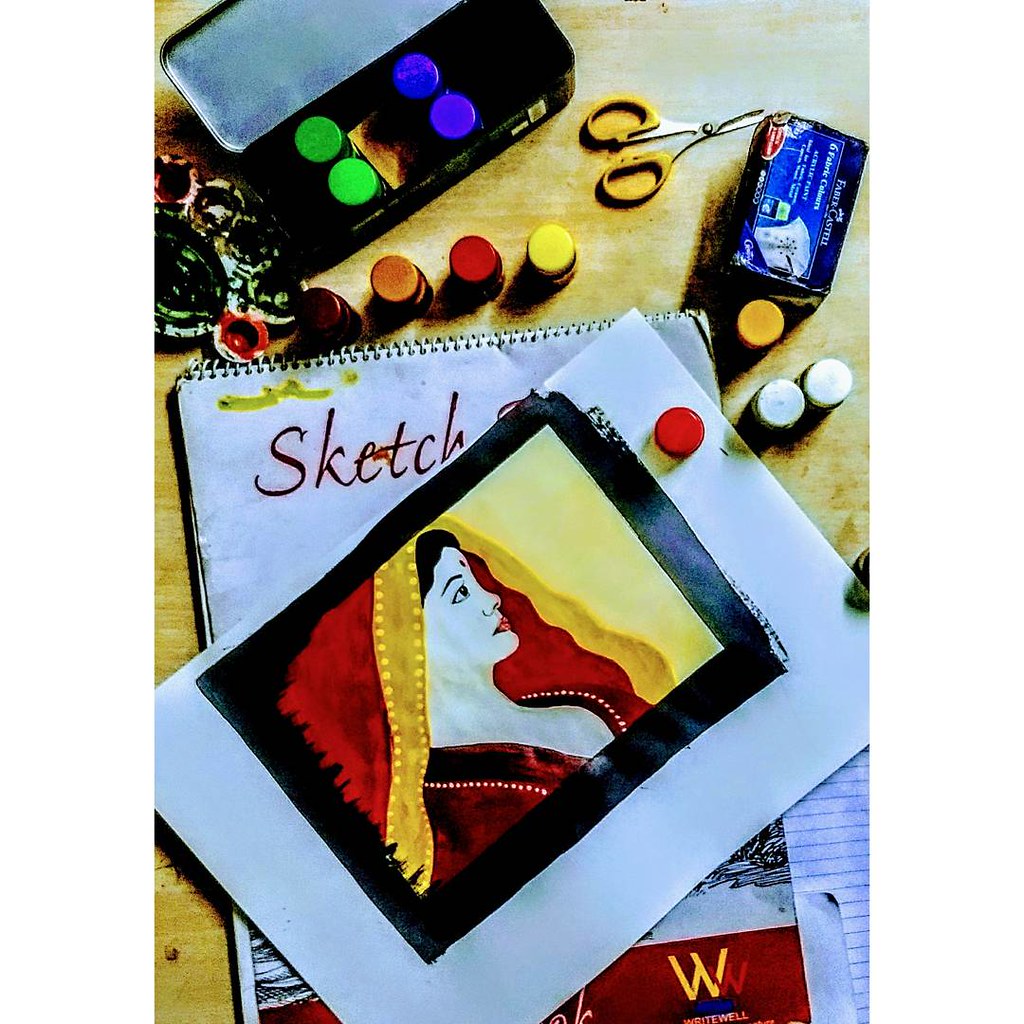This photo offers a detailed overhead view of an artist's workspace set on a light-colored wooden table. Central to the image is a sketch pad and several papers adorned with various artworks. Surrounding these are a multitude of small containers filled with paints in a vibrant array of colors, including red, yellow, orange, white, blue, green, and a dark red. A pair of small, orange scissors lies close by, next to a blue box with white lettering, though the text is indiscernible. In the upper left-hand corner, a metal container is flipped open, revealing its contents: numerous small bottles of paint. Situated to the left of this container is a paint tray, ready for mixing and blending colors during creative sessions. The composition of this workspace exudes inspiration and creativity, capturing the essence of an artist deeply immersed in their craft.